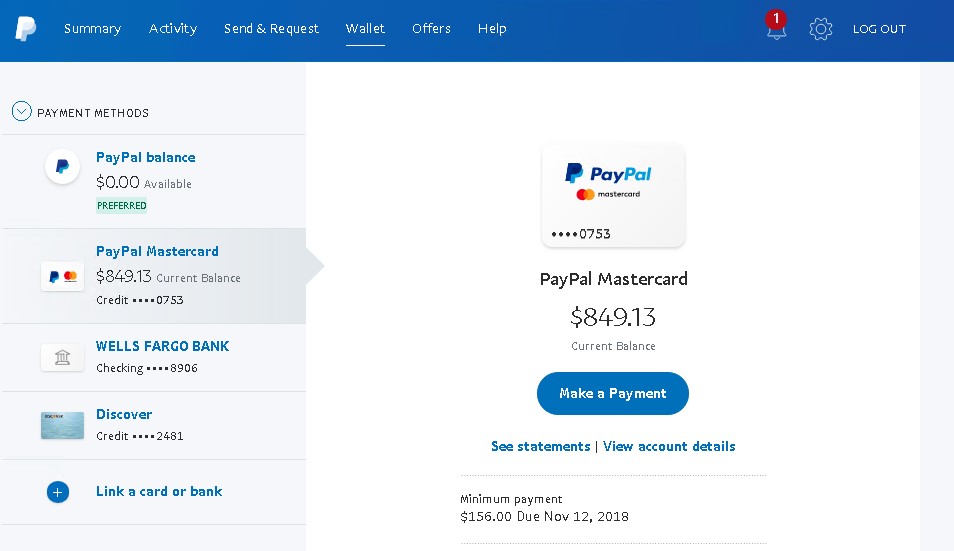**Website Overview: PayPal User Dashboard**

The user's PayPal dashboard is displayed with a blue header featuring a white "P" logo on the left. The navigation bar includes the following tabs: Summary, Activity, Send and Request, Wallet, Offers, and Help. A red notification icon with the number "1" indicates a new alert. Additionally, links for Settings and Logout are available.

Below the header, the "Payment Methods" section outlines the following details:

1. **PayPal Balance**: $0 Available (Preferred)
2. **PayPal MasterCard**: 
   - Current Balance: $849.13 
   - Card Ending: 0753
3. **Wells Fargo Bank Checking**
4. **Discover Credit Card**
5. A plus sign (+) indicating the option to link a new card or bank account.

To the right, the details of the PayPal MasterCard are highlighted:

- **Current Balance**: $849.13
- **Make a Payment**: Available option
- **See Statements**: Available option
- **View Account Details**: Available option
- **Minimum Payment Due**: $156 by November 12, 2018

No other details are present on the page.